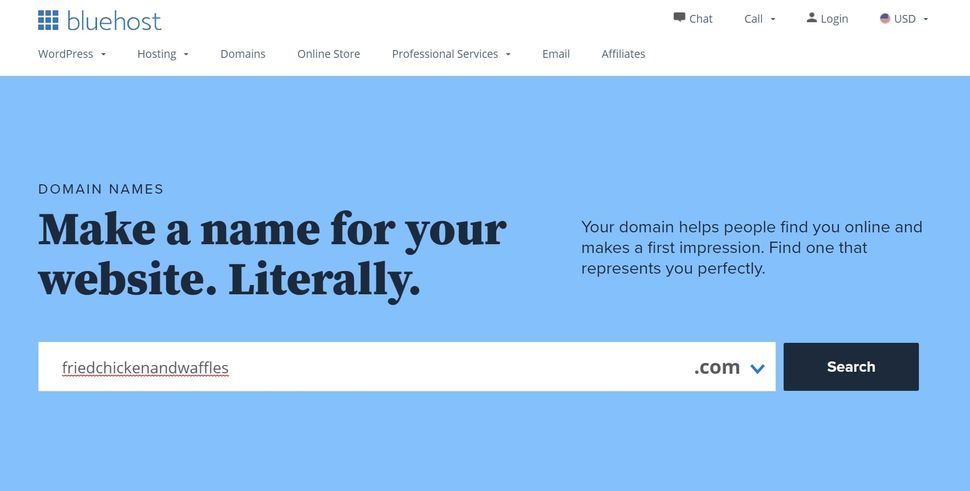The homepage of the Bluehost website features a clean and organized layout. At the very top, a white strip spans the width of the screen. On the furthest top left corner, there are nine blue blocks arranged in a 3x3 grid, resembling a simplified, one-dimensional Rubik's Cube. Next to these blocks, the word "Bluehost" is displayed in small caps.

On the far right of this white strip, options for "Chat," "Call," "Login," and the currently selected currency "USD" are listed. Below this header, a secondary navigation menu includes links labeled "WordPress," "Hosting," "Domains," "Online Store," "Professional Services," "Email," and "Affiliates."

The main section of the page features a very light, almost sky blue background. Prominently displayed at the top of this section is the phrase "Domain Names," written in small caps and dark blue font. Below that, in a bold and much larger font, the headline "Make a Name for Your Website" is prominently shown.

On the far right, a smaller font provides additional context: "Your domain helps people find you online and makes a first impression. Find one that represents you perfectly." Beneath this text is a search bar where users can input their desired domain name. In this instance, the user has typed "friedchickenandwaffles.com," which is underlined. Adjacent to the search bar, a dark blue button with the word "Search" written in white is ready to be clicked.